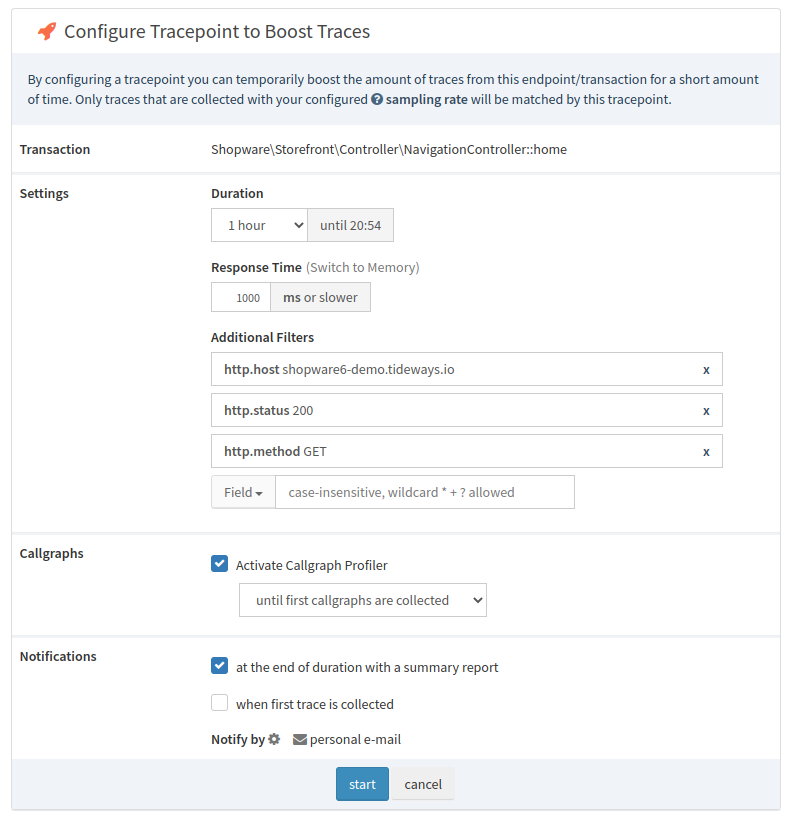The image depicts a detailed webpage interface for configuring a trace point to boost traces. At the top is an orange rocket icon accompanied by the text, "Configure Trace Point to Boost Traces." Beneath this, on a blue background, there is an explanatory message, "By configuring a trace point, you can temporarily boost the amount of traces from this endpoint/transaction for a short amount of time. Any traces that are collected with your configured sample rate will be matched by this trace point."

The webpage features a "Transaction" section listing the current transaction path as "Shopware/Storefront/Controller/NavigationController" with the specific page "Home." In the "Settings" section, the duration is set to "1 hour until 20:54," and the response time condition is "1000 ms or slower."

An "Additional Filter" section offers more parameters, such as host details related to Shopware and a status code defaulted to 200. There's also a section for "Call Graphs" with an activated checkbox labeled, "Activate call graph profiler until first call graphs are collected." 

The "Notifications" section includes an option to receive a summary report at the end of the duration, marked with a blue checkmark. Another box for receiving notifications when the first trace is collected is present but unchecked. 

Towards the bottom, there's a statement in black, "Notify by settings or personal email," with two main action buttons: a blue "Start" button and a gray "Cancel" button. Most of the webpage is set against a white background.